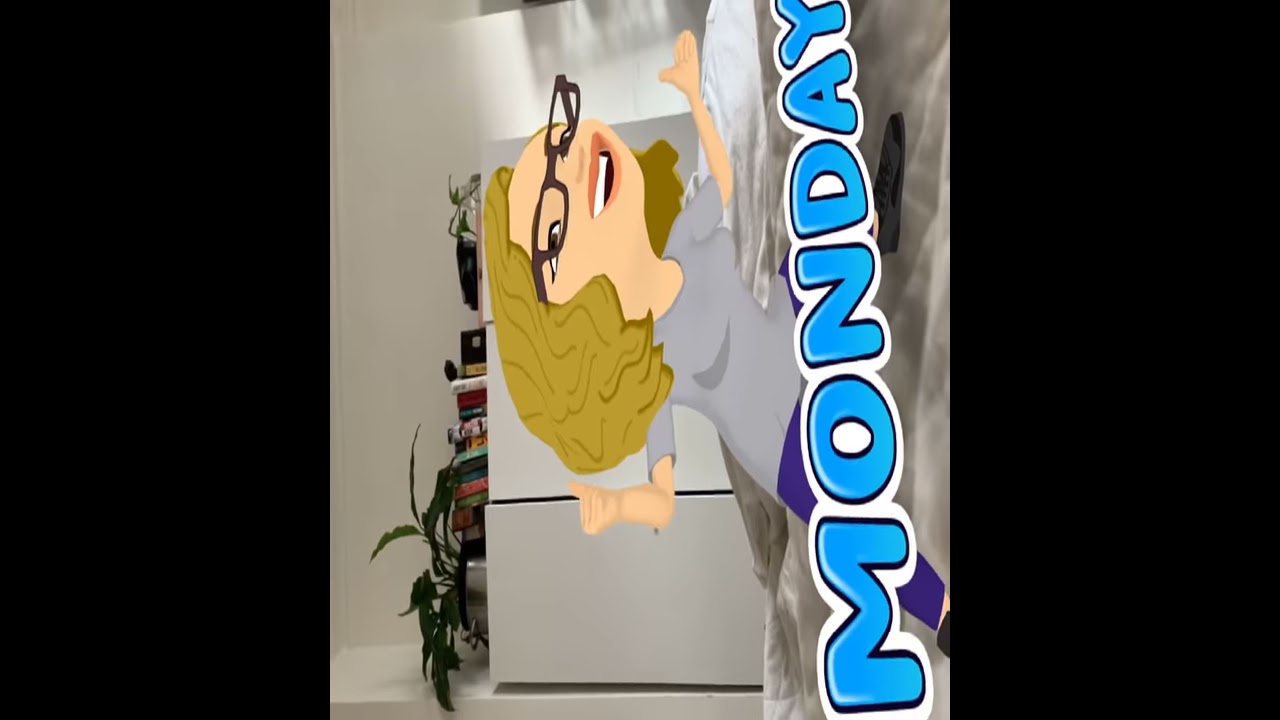The sideways image presents a slightly disorienting scene set on a bed with a wrinkled white blanket. Behind the bed, a white cabinet, which resembles a bookcase, is visible with various books lined neatly on top and a broadleaf plant in a metal pot. Adding a touch of greenery. Dominating the foreground, a digitally overlaid cartoon woman with short blonde hair, black glasses, brown eyes, and a cheerful smile stands prominently. She is dressed in a gray blouse, blue pants, and black shoes, with her arms enthusiastically raised. Curved, bubbly, bright turquoise letters, outlined first in black and then in white, spell out "Monday" vertically to her right, contributing to the playful and vibrant tone of the image.